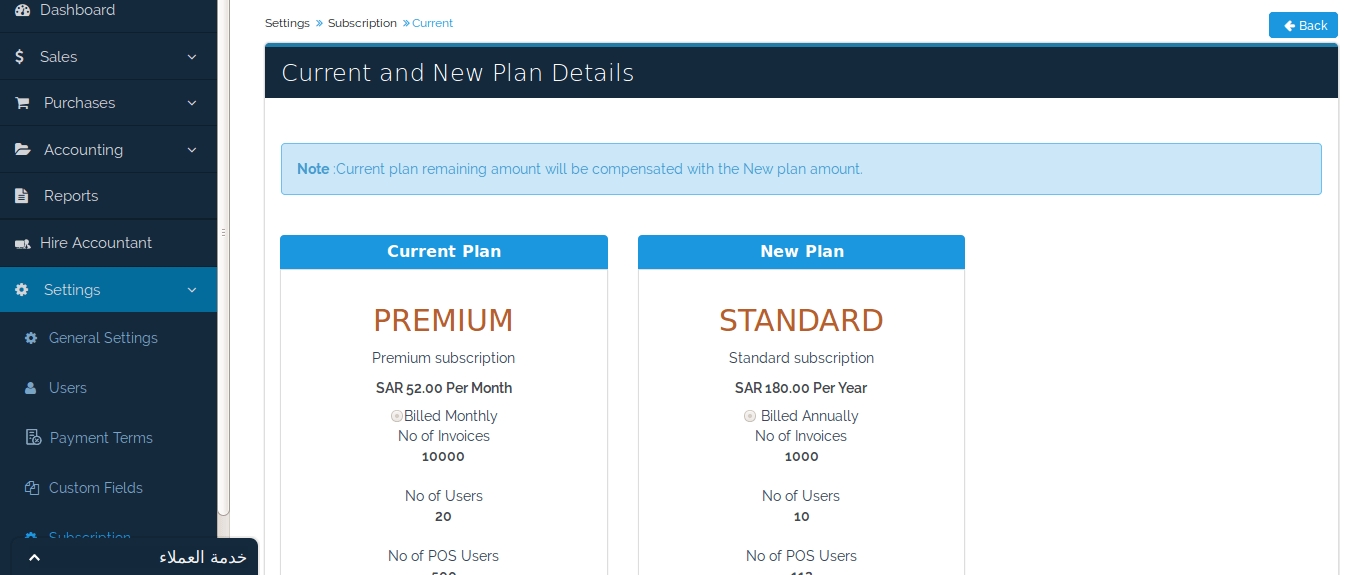**Detailed Caption:**

The screenshot depicts a user interface of a software application. On the left-hand side of the screen, a sidebar menu lists various navigation options including "Dashboard," "Sales," "Purchases," "Accounting," "Reports," "Hire Accountant," "Settings," "General Settings," "Users," "Payment Terms," and "Custom Fields."

On the right-hand side, the interface shows detailed settings related to the user's subscription plan. It provides options to view the current subscription, compare with a new plan, and navigate back. 

The current plan is labeled as "Premium," costing SAR 52 per month, billed monthly. This plan allows for the creation of up to 10,000 invoices and supports 20 users. 

The new plan, referred to as "Standard," is priced at SAR 180 per year, billed annually, allowing for up to 1,000 invoices and supporting 10 users. There is a special note indicating that the remaining amount of the current plan will be compensated with the new plan amount upon subscription change.

The screen captures an important moment where the user is comparing the features and costs of the two subscription plans before making a decision.